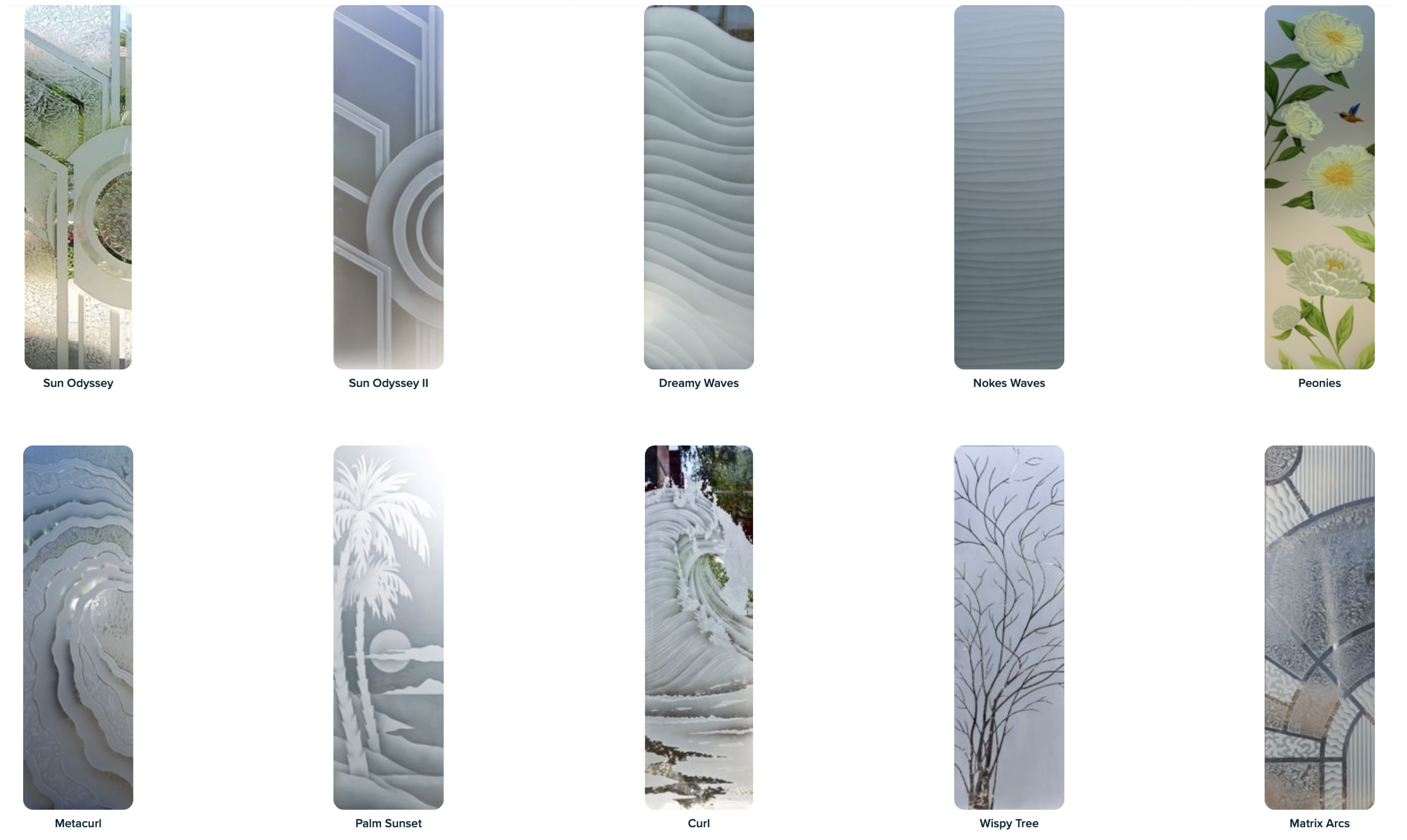In this image, there is a collection of ten distinct smaller images, each with unique visual elements and titles. 

1. **Sun Odyssey**: This image features a white, round background adorned with tall, white stripes that resemble reflections on mirrors.
2. **Sun Odyssey 2**: Set against a gray background, this image showcases a nearly circular floral pattern in the center, flanked by white lines on either side.
3. **Dreamy Waves**: Here, elegant white wave patterns emerge, conveying a serene and fluid motion.
4. **Notes Waves**: This image presents modest, gray-toned lines that create a minimalist and rhythmic pattern, reminiscent of gentle waves.
5. **Peonies**: A depiction of delicate white peonies, accompanied by lush green leaves, highlighting the beauty of these flowers.
6. **Palm Sunset**: An image capturing the tranquil silhouette of a palm tree against a colorful, warm sunset sky.
7. **Curl**: Featuring a singular curl or spiral, this image emphasizes simple, graceful lines and curvature.
8. **Waspie Tree**: This intriguing image may depict a unique tree, potentially characterized by distinct or wasp-like attributes.
9. **Pretty Mosaic**: A visually appealing mosaic, composed of various colors and shapes, creating a captivating and intricate design.
10. **[Unspecified Image]**: The description ends without detailing the tenth image, leaving it open to interpretation or unobserved in the given narrative.